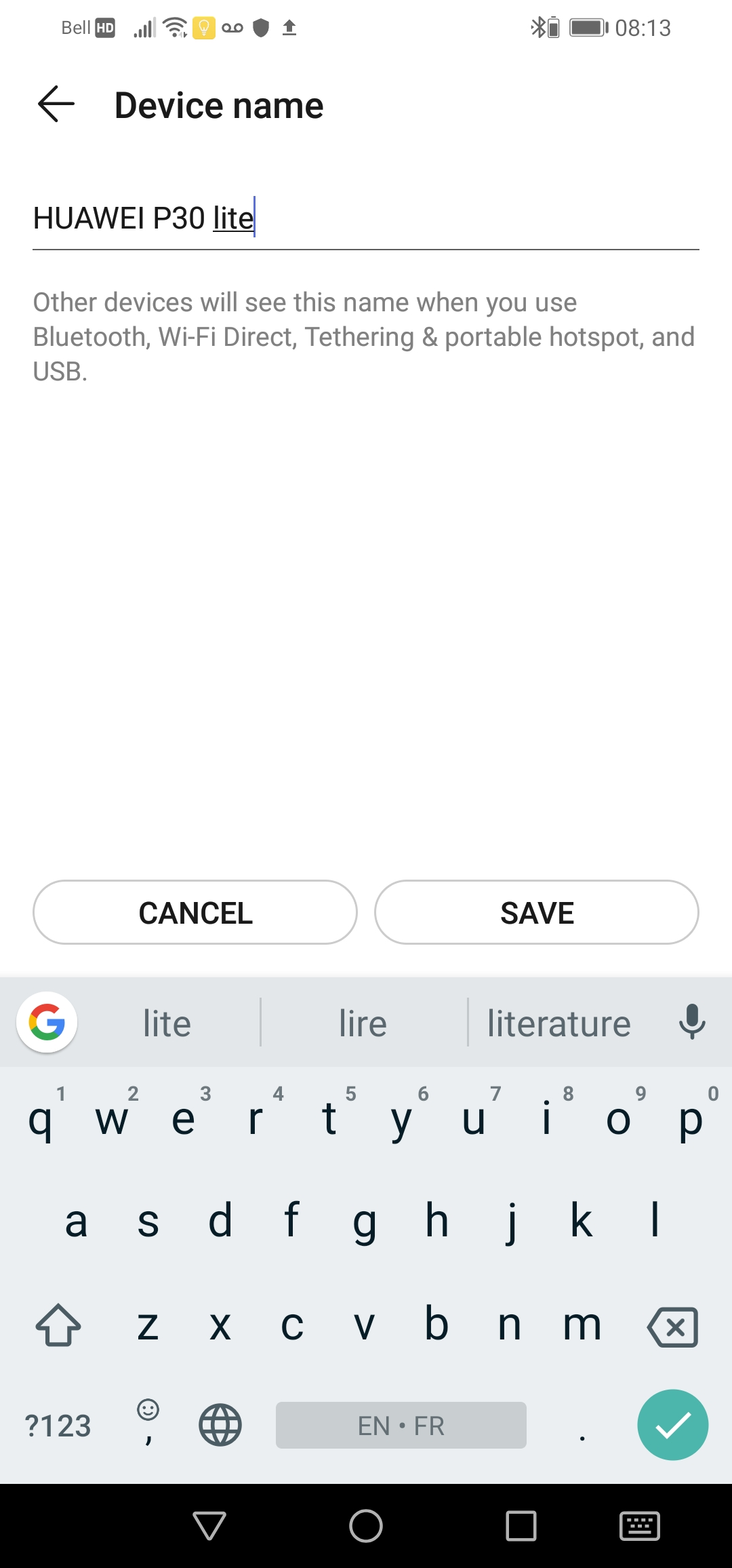The image displays a detailed digital interface with various icons and text elements organized across the screen. 

At the top, there are several status symbols: a bell icon, an indistinct grey square with unclear letters, a signal strength bar graph with increasing line heights moving to the right, a Wi-Fi symbol, a yellow square containing a white shape, two connected circles, an upside-down teardrop shape, and an upward-pointing arrow. 

On the left-hand side of the screen, there are two triangles with a partial triangle below them, a vertical battery icon, and a horizontal battery icon, followed by the number "813". Below this, there's a leftward-pointing arrow alongside text reading "Device Name," followed by the name "HUAWEI P30 LIGHT" with a blue line after "LIGHT". Beneath this, there's grey text stating: "Other devices will see this name when you use Bluetooth, Wi-Fi Direct, Tethering & Portable Hotspot, and USB."

Further down, there are two rounded rectangles. The first one says "Cancel," and the second says "Save."

In a grey rectangle below, there is a white circle featuring the Google "G". Adjacent to this, there are lines of text reading "Light," "Liar," and "Literature." To the side, there's a microphone symbol. Below this, there's a keyboard layout with "?123," an icon resembling a smiley face with a notch underneath, a globe icon, and a grey rectangle with "EN.FR" written on it. This area also features a blue-green circle with a checkmark, and a black rectangle containing a downward-pointing triangle, a circle, a square, and another keyboard symbol.

The overall display provides a snapshot of a smartphone's user interface, illustrating various functional icons, device status indicators, and options for connectivity and text input.